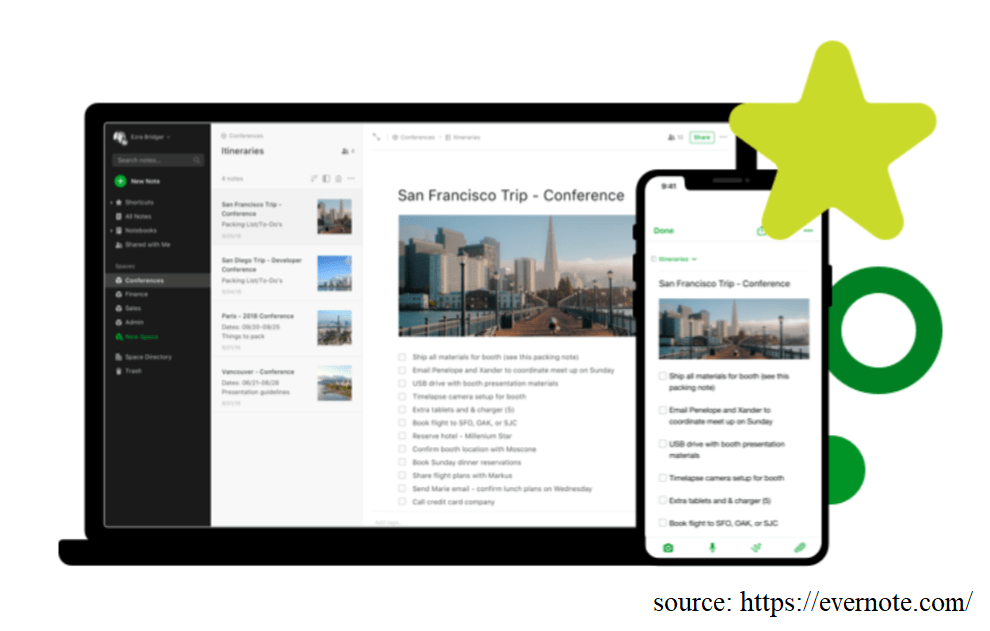A stock photo showcases a laptop and a mobile phone placed side by side. The entire laptop is visible in the image, including its casing, with a program displayed on its screen. To the right of the laptop lies the mobile phone. The mobile phone's volume button is located on the left side, while its power button is on the right. A green star is positioned above the devices at their corner. To the right of the mobile phone, there is a hollow circle outlined in green. 

On the laptop screen, the program features a black sidebar with the remainder of the webpage in a lighter color. The displayed name on the website reads "San Francisco Trip Conference," accompanied by a picture of San Francisco. The mobile phone screen shows the same webpage, albeit in a more condensed format also titled "San Francisco Trip Conference," with checkboxes situated below the San Francisco image on both devices. A source line at the bottom right of the image reads, "source https://evernote.com."